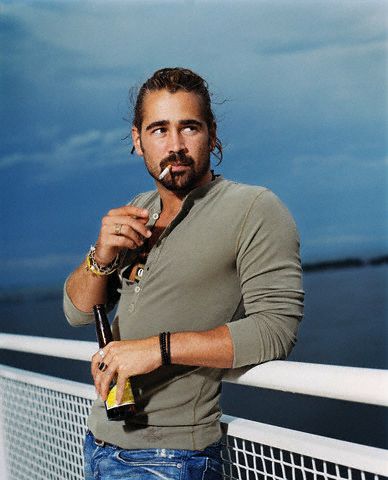In the image, taken outdoors during the early evening, a man stands in front of a white mesh fence, likely on a ship or a bridge. The background features a darkening blue sky filled with clouds, with the ocean visible in the far right corner and trees in the distance. The man, who resembles a known actor, is leaning against the railing with his elbow, appearing muscular and casually dressed in a buttoned-down grey sweater and blue jeans. He's smoking a cigarette, holding it with his right hand close to his mouth, and also holding a bottle of beer in his left hand. The man wears multiple pieces of jewelry: black bracelets on his left wrist, chains on his right, and rings on several fingers. His gaze is directed slightly upwards and to the right, looking at something or someone in the distance.